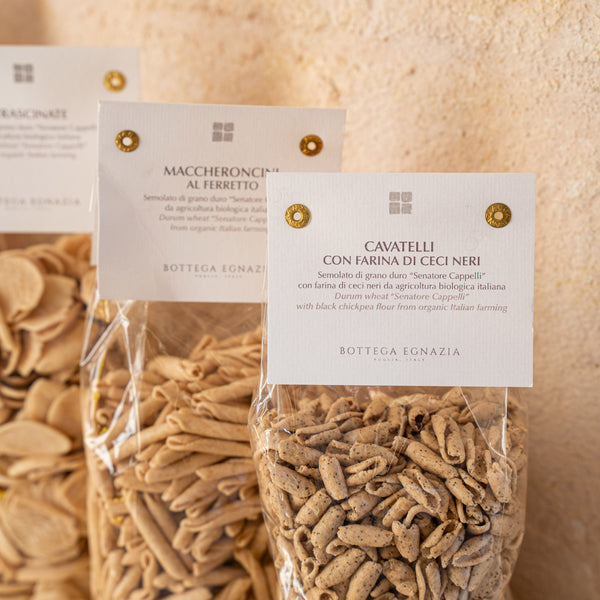The image depicts three vertically-aligned, clear plastic bags of pasta against a light brown stone wall. Each bag is progressively taller and positioned slightly to the left, allowing for visibility of all three. The closest bag contains curved rectangular pasta pieces labeled "Cavatelli Con Farina di Cecchianeri" and is attached to the bag via a white label with brass rivets. The second bag, which is taller and further left, encases cylindrical pasta labeled "Maccheroncini Al Farito." The final and tallest bag has small disc-shaped pasta with an unreadable, blurred label. All bags belong to the brand Bottega Ignazia and suggest a premium quality, likely corresponding to higher prices. The pasta appears dried, intended for reconstitution through cooking.